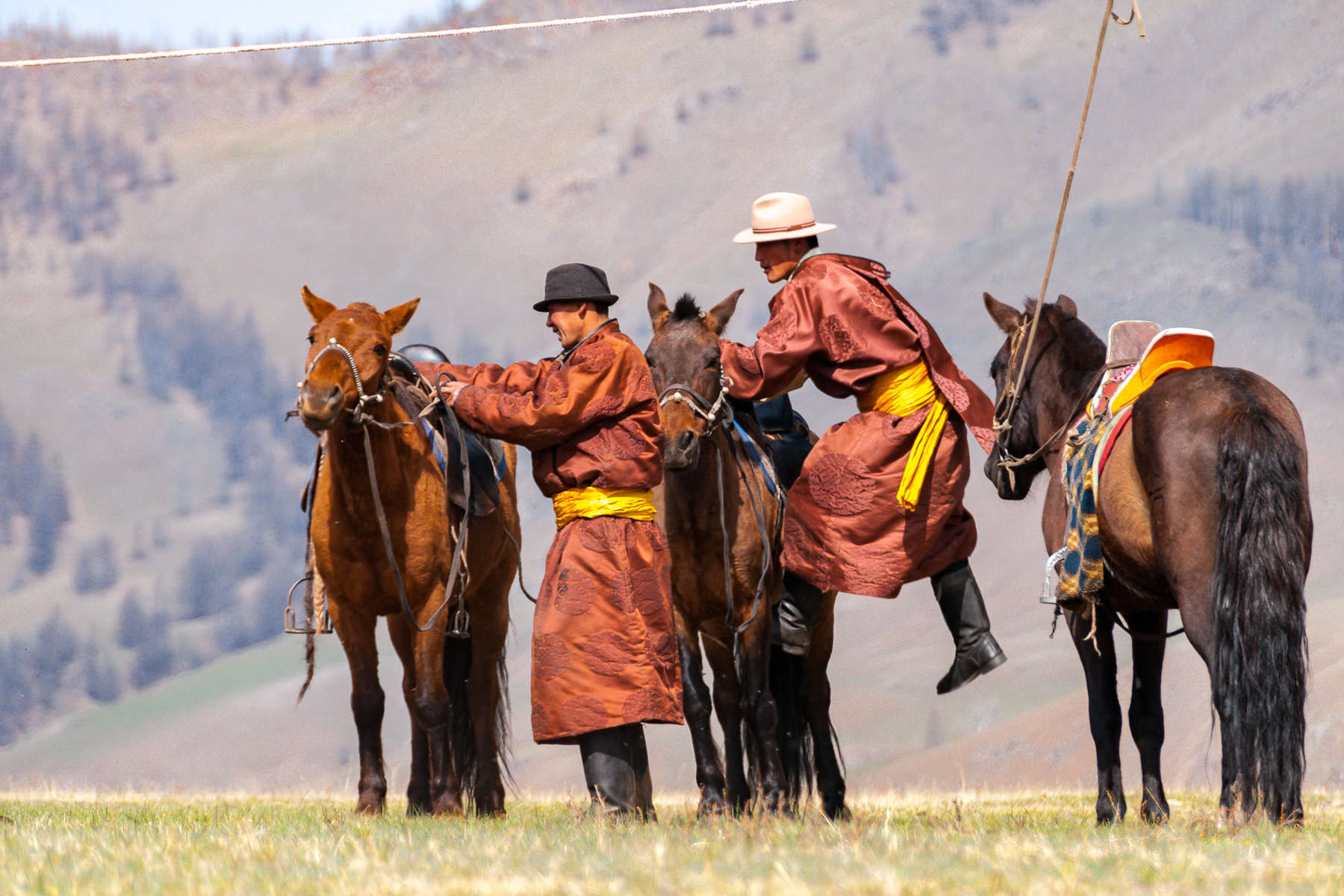In the image, two men clad in distinctive russet-brown robes that fall past their knees, belted with bright yellow sashes, are engaging with three small brown horses. One man, mid-air, is about to mount his horse, while the other is fixing the saddlebags. These outfits, along with their fedora-style hats, suggest a unique cultural attire, possibly indicating a region like Peru or parts of China. The horses, two dark brown and one reddish-brown, have matching yellow accents on their saddles, echoing the men’s sashes. The setting is a grassy area bordered by dry, mountainous terrain, with a high depth of field that blurs the distant mountains. A taut rope, barely visible, runs across the top of the image, possibly strung between two unseen trees, to which the horses may be tied during a pause in their journey. The overall scene suggests that the men are preparing for a trip, as they meticulously ready themselves and their horses, all set against a picturesque backdrop.